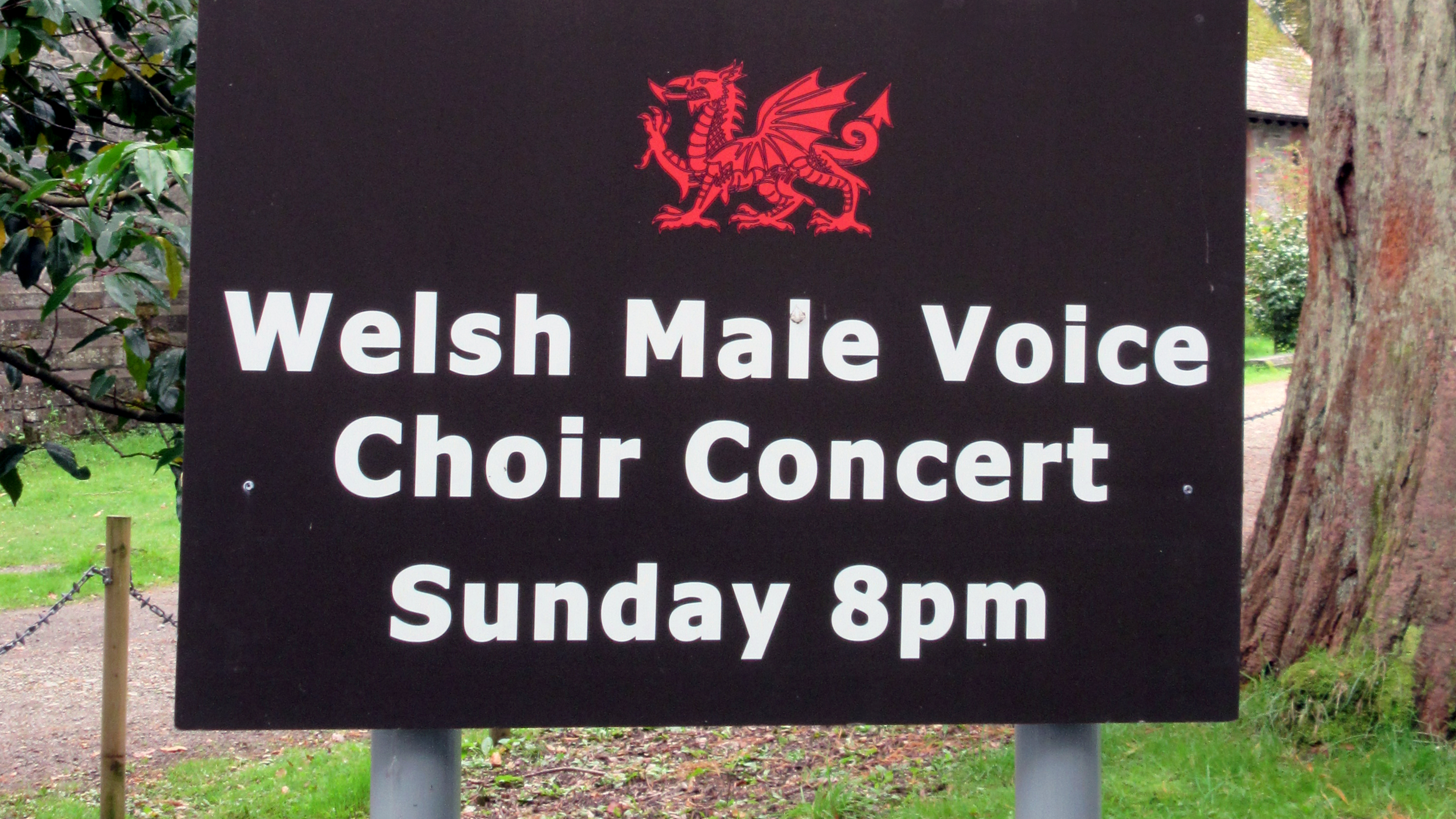The photograph captures an outdoor scene centered around a large black sign with white text that reads "Welsh Male Voice Choir Concert, Sunday, 8pm." Dominating the top of the sign is a detailed red dragon illustration, its tongue sticking out, raising its right arm, with an arrow-shaped coiled tail, and outstretched wings. The sign is securely mounted to the ground with two thick, gray metal poles.

The setting includes a gravel path adjacent to the sign, with a wood and wire fence running parallel to it in the background. To the left of the sign are posts with chains designed to prevent foot traffic on grassy areas. Trees form part of the backdrop, with a particularly notable tree trunk with moss located on the far right, along with patches of grass. The background also reveals a glimpse of a brick building partially obscured by bushes. Additional details include a green and brown tree to the left and a reddish-gray tree trunk on the right side of the image.